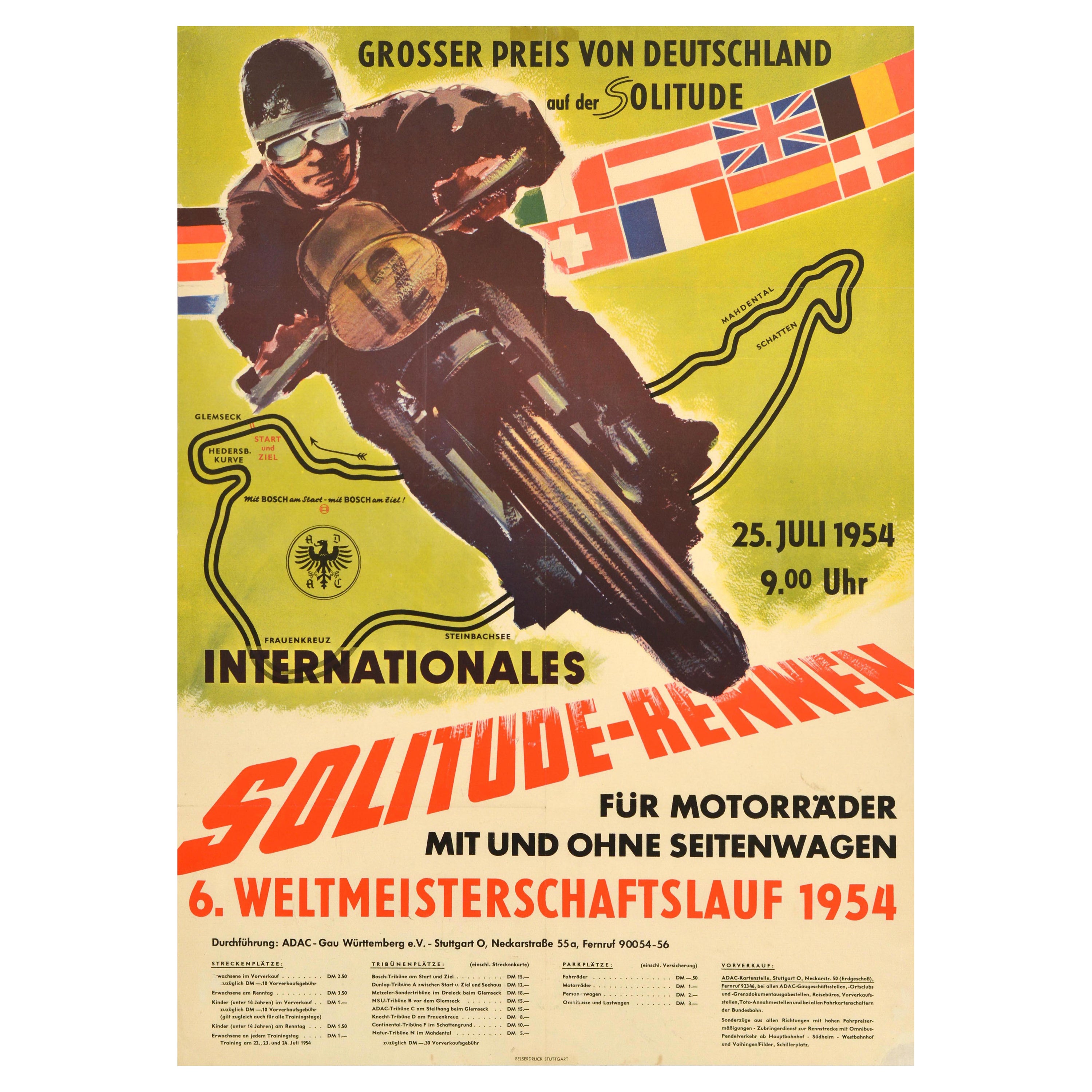This vertical poster, appearing to be an advertisement for motorcycle racing, prominently features the title "Grosser Preis von Deutschland auf der Solitude" at the top. The primary image showcases a motorcyclist, dressed in brown gear with a black helmet and white or gray sunglasses, riding a sharply tilted motorcycle labeled with the number 12. His head is in the top left corner while the front wheel points diagonally to the right. The poster, likely dated July 25, 1954, as indicated by "25 JULI 1954" and "9.00 UHR" at the bottom, includes various German texts, with "Solitude Rennen" in bold red letters near the middle. A banner of international flags stretches across the upper section, and behind the motorcyclist, there appears to be an outline resembling a map, potentially indicating a race route. The small text at the bottom could be the names of the racers.